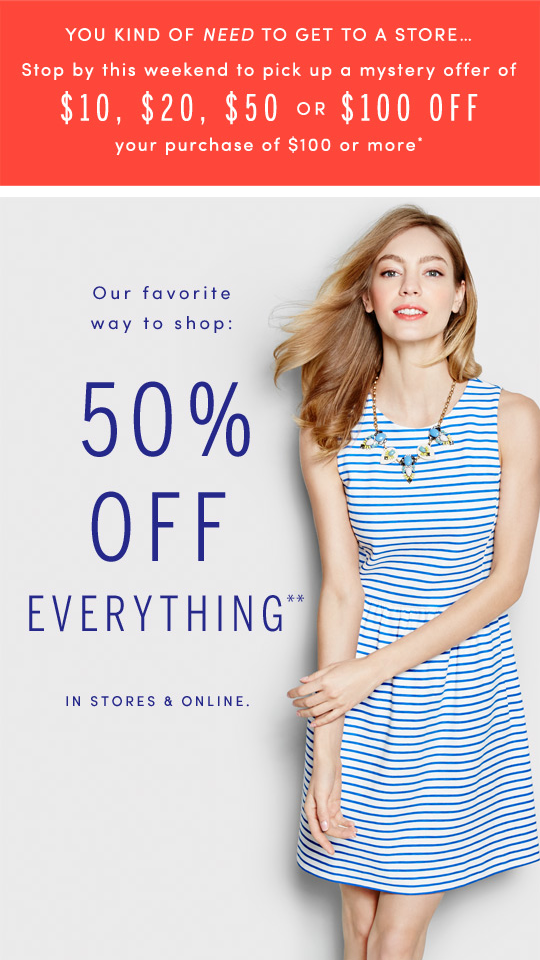In this promotional image, the top portion features a rectangle with a striking red background, adorned with white text. The message reads, "You kind of need to get to a store... stop by this weekend to pick up a mystery offer of $10, $20, $50, or $100 off your purchase of $100 or more."

Below this, in the larger, grayish background section of the image, a stylish woman captures attention on the right side. She gazes directly into the camera, exuding confidence in a white dress adorned with blue horizontal stripes. She accessorizes with a gold-colored necklace, featuring five pieces of jewelry in shades of white and blue, complementing her light brown hair, pink lipstick, and bluish eyes. To her left, bold dark blue text proclaims, "Our favorite way to shop: 50% off everything in stores and online." This engaging visual and text arrangement effectively promotes a significant sale and mystery discount offer, enticing viewers to visit the store.